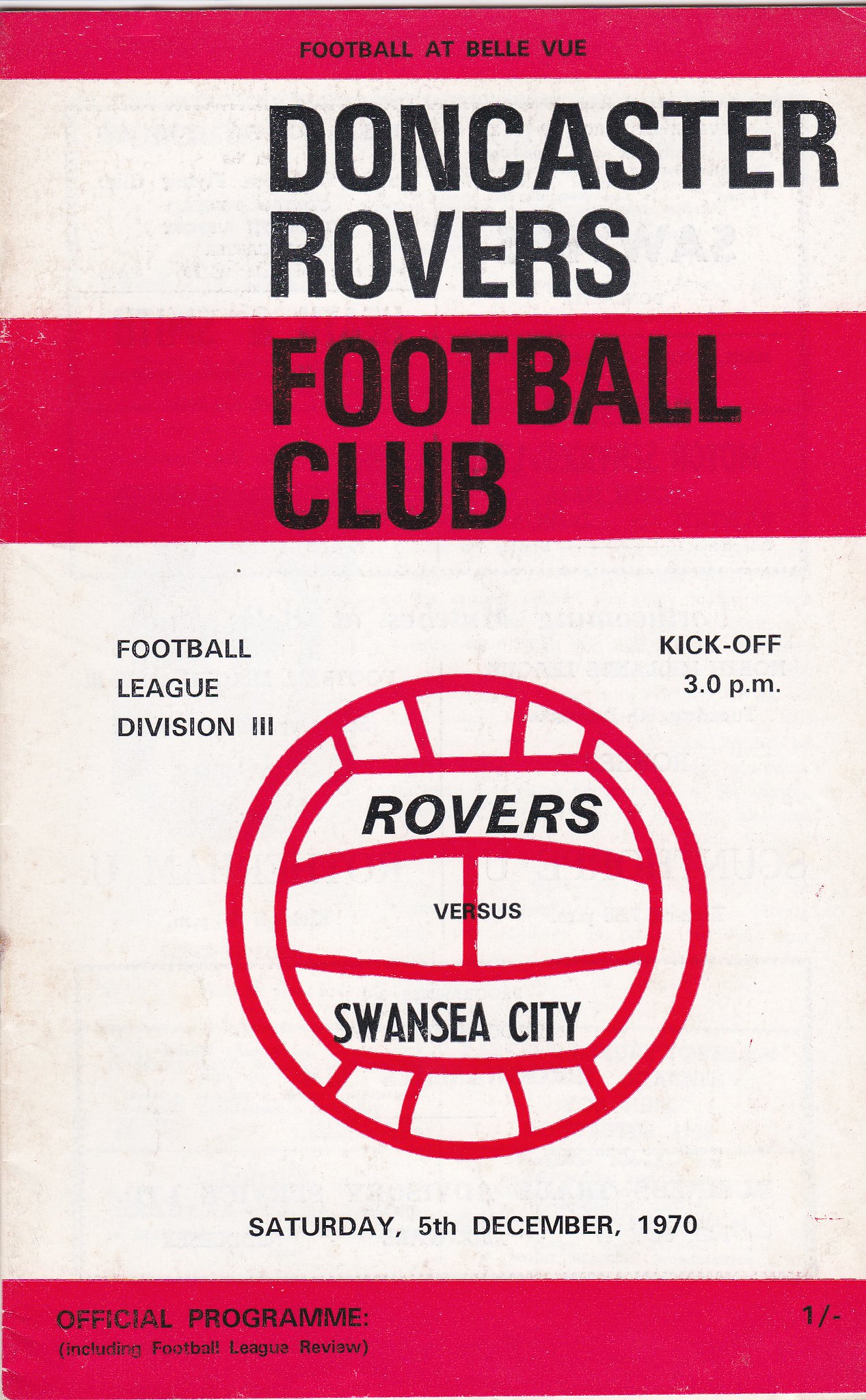This is an official program for a British football match between Doncaster Rovers and Swansea City in the Football League Division 3. The cover features black text over white and red stripes, with a central illustration of a soccer ball. Notably, the program details the match scheduled for 3 p.m. on Saturday, December 5, 1970. The text "Rovers versus Swansea City" is prominently displayed, alongside "Official Program" and an inclusion of the "Football League Review." The colors on the program have a faded, worn appearance, indicative of its vintage nature.